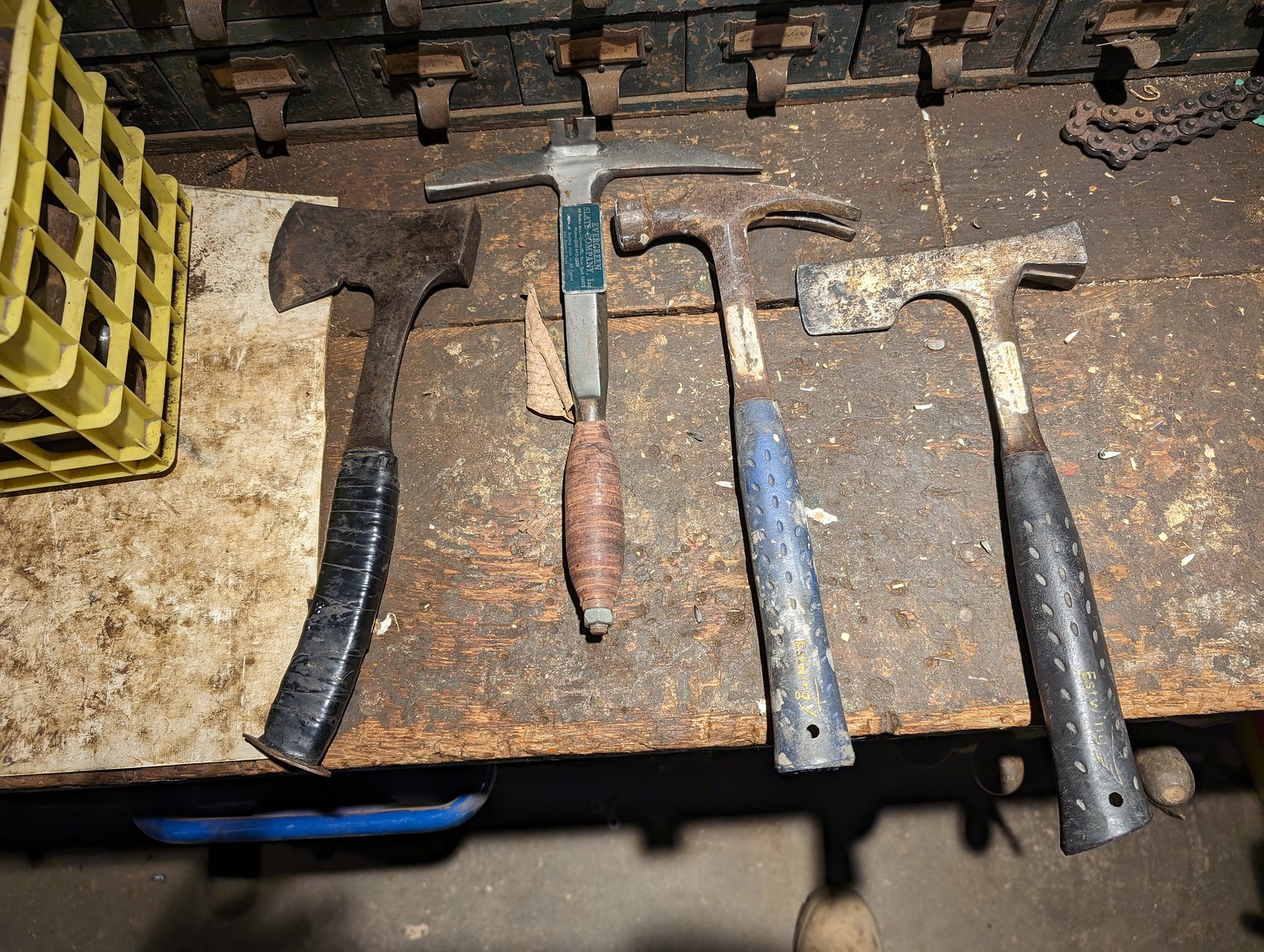The photograph depicts a cluttered and well-worn workspace, possibly a workshop. Central to the scene is a heavily-used, multi-colored metal table with evident grime, featuring both white and brass-colored dirty surfaces. Atop the table on the left, there’s a yellow milk basket, typically used for holding glass bottles. Below the table to the left, there’s a blue, standalone utility trolley. Scattered across the table are several old and rusty tools: a hatchet with a taped black handle and a dirty brown metal head, a pickaxe with a thick orange handle and metallic silver head, a hammer with a blue handle and a rusty brown head, and a multi-functional tool combining a hammer and hatchet, characterized by a black handle and a white, rusted top. A bicycle chain is also noticeable on the table. The floor beneath, visible at the bottom of the image, is composed of black concrete, showing the shadows cast by the various objects.